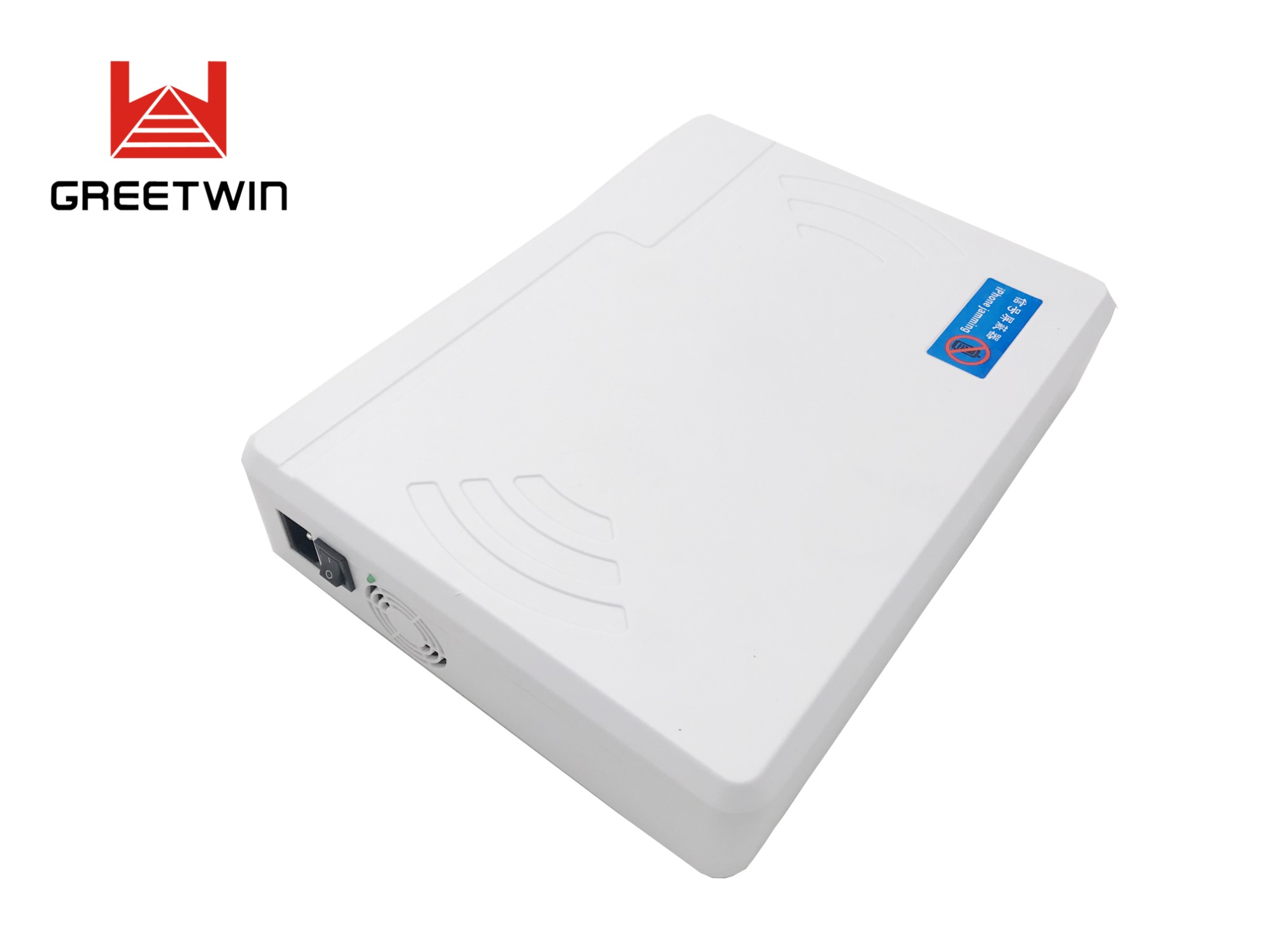This image depicts a white electronic device, possibly a wireless router or Bluetooth adapter, manufactured by GREETWIN. The device appears as a small, flat, square box with a clean, scratch-free surface. Positioned on the top left is the GREETWIN logo, which features a design resembling white railroad tracks on a red background. Accompanying this, there are symbols similar to arcs or swooshes, potentially indicating signal transmission capabilities.

A blue rectangular sticker with unreadable text is affixed to the top, featuring a noticeable cross mark. On the side, there's a black power switch, situated next to an Ethernet port for connectivity and a vent cut-out designed to keep the device cool. The overall design and ports suggest this device is intended to enhance or provide wireless communication, possibly transforming a computer into a Bluetooth or Wi-Fi-enabled device.